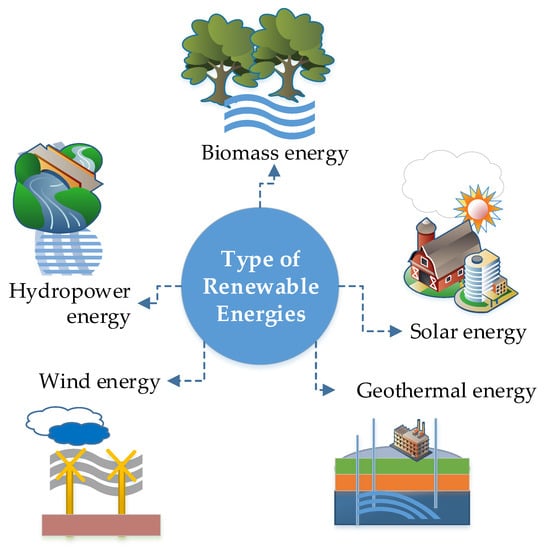The chart visually represents five types of renewable energies with distinct illustrations and color codes. In the center, a blue circle with white text reads "Types of Renewable Energies," connecting to each energy type via blue dotted arrows. 

In the lower right, geothermal energy is illustrated with a power plant on gray land, beneath green, orange, and blue layers, suggesting geothermal heat extraction. The bottom left depicts wind energy with yellow wind turbines on a pink surface, accompanied by three wavy gray lines symbolizing wind. 

On the left, hydropower energy features what appears to be a stream in green and gray hues, with white lines depicting water movement and blue and white cross-touch lines indicating hydropower generation. 

At the top, biomass energy is represented by two green trees above three blue wavy lines, indicating organic material processing. 

Finally, to the right, solar energy is shown with a bright sun emitting orange, yellow, and white rays, hovering over a farmhouse with a silo and another multi-level building, possibly for solar energy processing, amid white cloud accents. The entire image is detailed with black text outside the circle and sections highlighted in colors like green, yellow, orange, blue, and black.